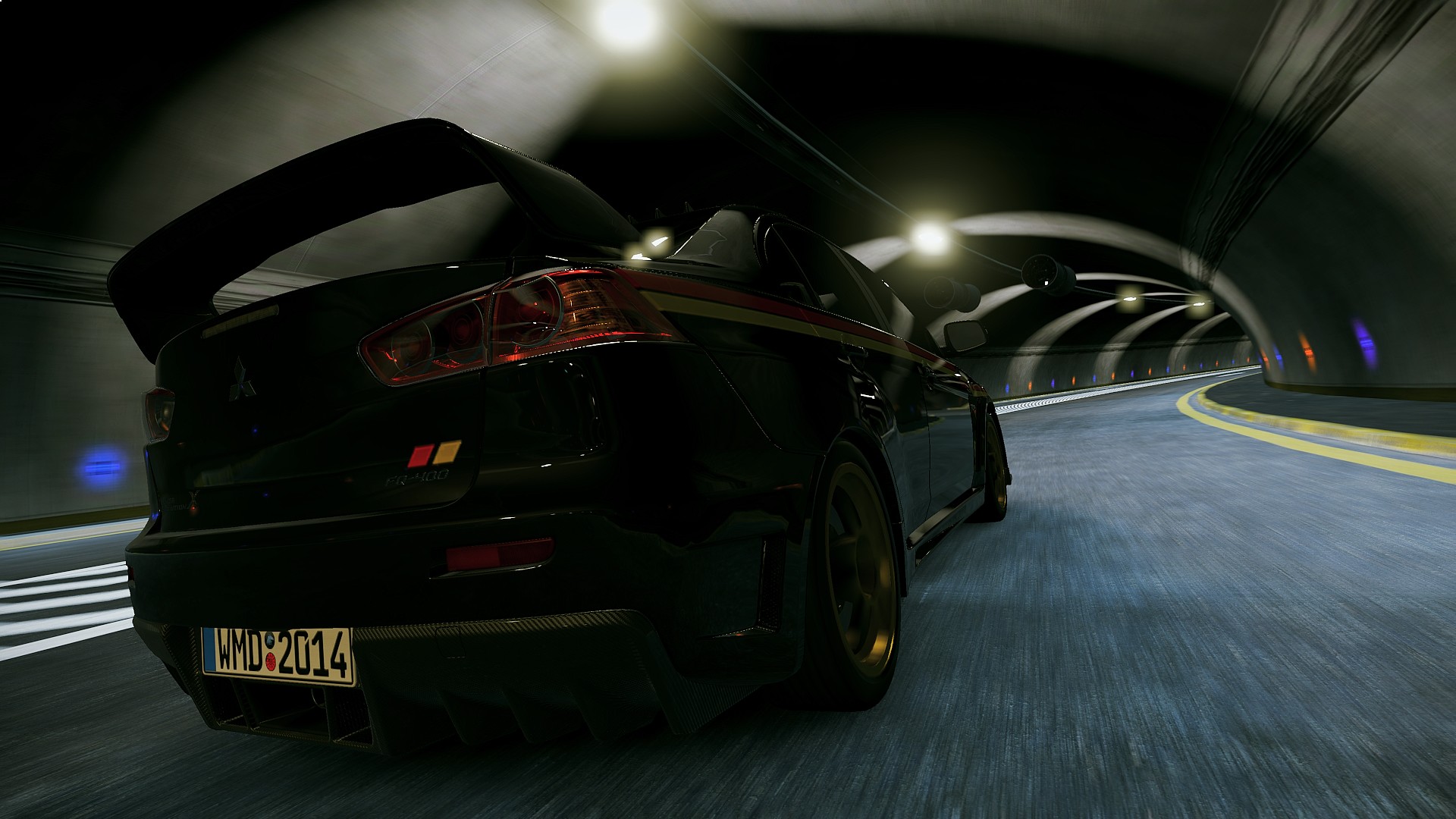The image showcases a sleek, black sports car with a black spoiler, captured from behind as it speeds through a modern gray tunnel. The composition is action-oriented and employs a wide-angle lens, emphasizing a dramatic sheen and a sense of motion. The car, potentially a Mitsubishi, features distinctive dark green and red stripes along its right side, just below the window. A white license plate with the text "WMD2014" is visible on the back. The tunnel is lined with lights on its ceiling, and the asphalt road, painted with various lines, curves to the right in the upper portion of the image. The scene exudes a slightly surreal, possibly 3D-rendered quality, intensifying the impression of high-speed movement.